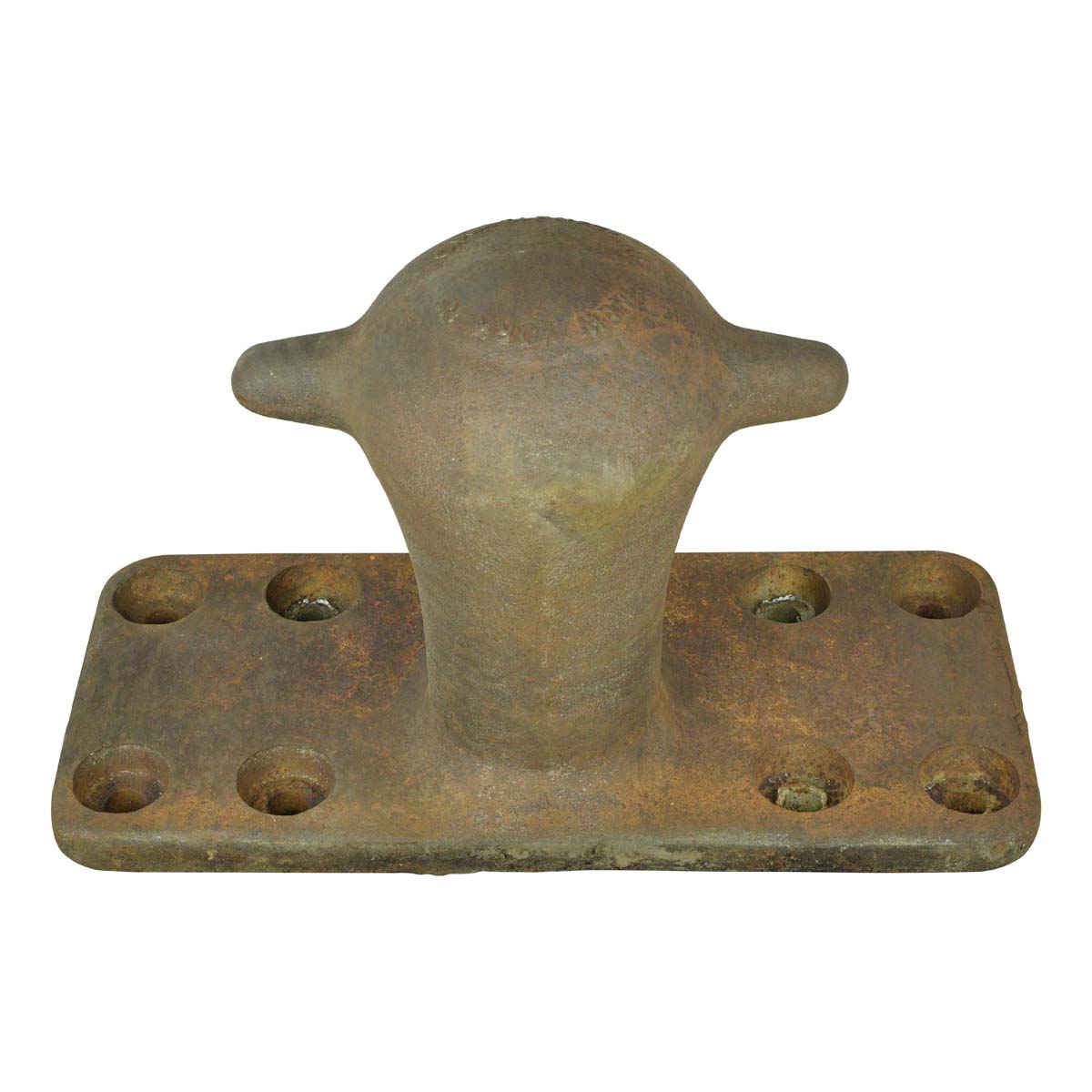The photograph depicts a large, rusted metal boat cleat, useful for tying boats to a dock. The cleat features a rectangular base, peppered with eight holes—four on each side for bolting the cleat securely to a surface. Protruding from the center of this base is a large, bulbous structure that expands at the top. From this central bulb, two rounded, ear-like handles extend horizontally, creating a T-shaped appearance. This entire object is significantly weathered, with a brownish hue indicating its age and extensive use. Decorative raised text encircles the top of the bulb, with part of it discernibly reading "New York," though the rest is obscured. This functional piece of maritime hardware evidently serves the purpose of anchoring boats securely to piers or docks.